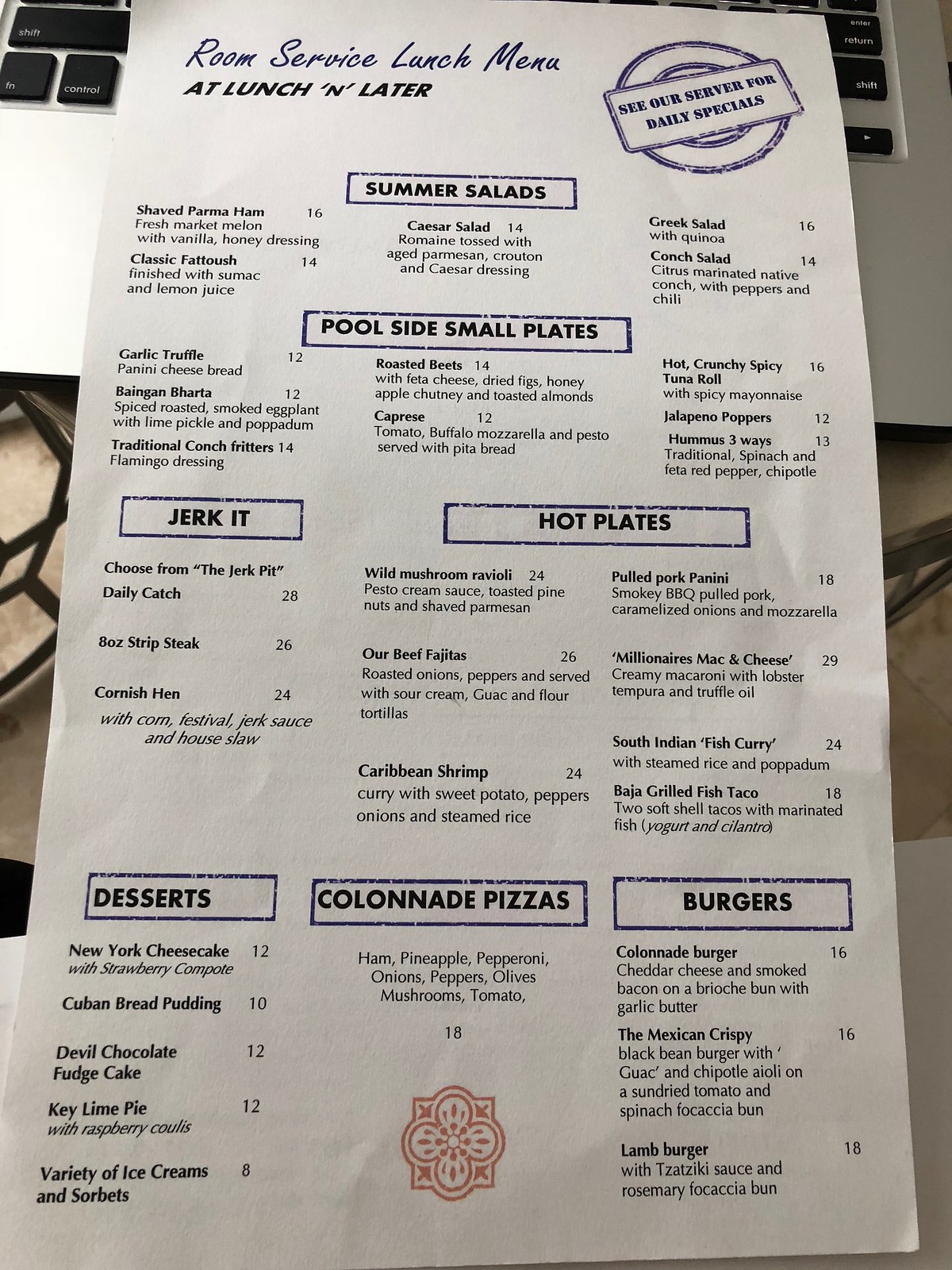The image showcases a detailed room service menu in black and white, placed over a silver laptop keyboard with black keys, and a brownish wooden desk beneath. On the left and right sides of the desk, there's a small metal structure, and at the bottom, a white piece of paper is partially visible under the menu. The menu’s layout is enhanced with purple accents, most notably around the headlines of each section, emphasizing their importance. 

At the top of the menu, in purple text, "Room Service Lunch Menu" is prominently displayed. Adjacent to it, a message in purple text against a purple plate-shaped background reads, "Ask your server for daily specials." Under the header, the first section titled "Summer Salads" listed within a purple-bordered box, features options such as shaved Parma ham, Caesar salad, classic fatoush, Greek salad, and conch salad.

Following that, the "Eat Poolside – Small Plates" section offers choices like garlic truffle, bang bang bar tuck, traditional conch fritters, roasted beets, caprese, hot crunchy spicy tuna roll, jalapeno poppers, and hummus three ways. Other menu categories include "Jerk It," "Hot Plates," "Desserts," "Colonnade Pizzas," and "Burgers."

At the bottom of the menu, there is an elegant red and white lotus pattern image enclosed in a square, further outlined with a red border that frames the entire menu, adding a touch of vibrant color to the overall monochrome design.